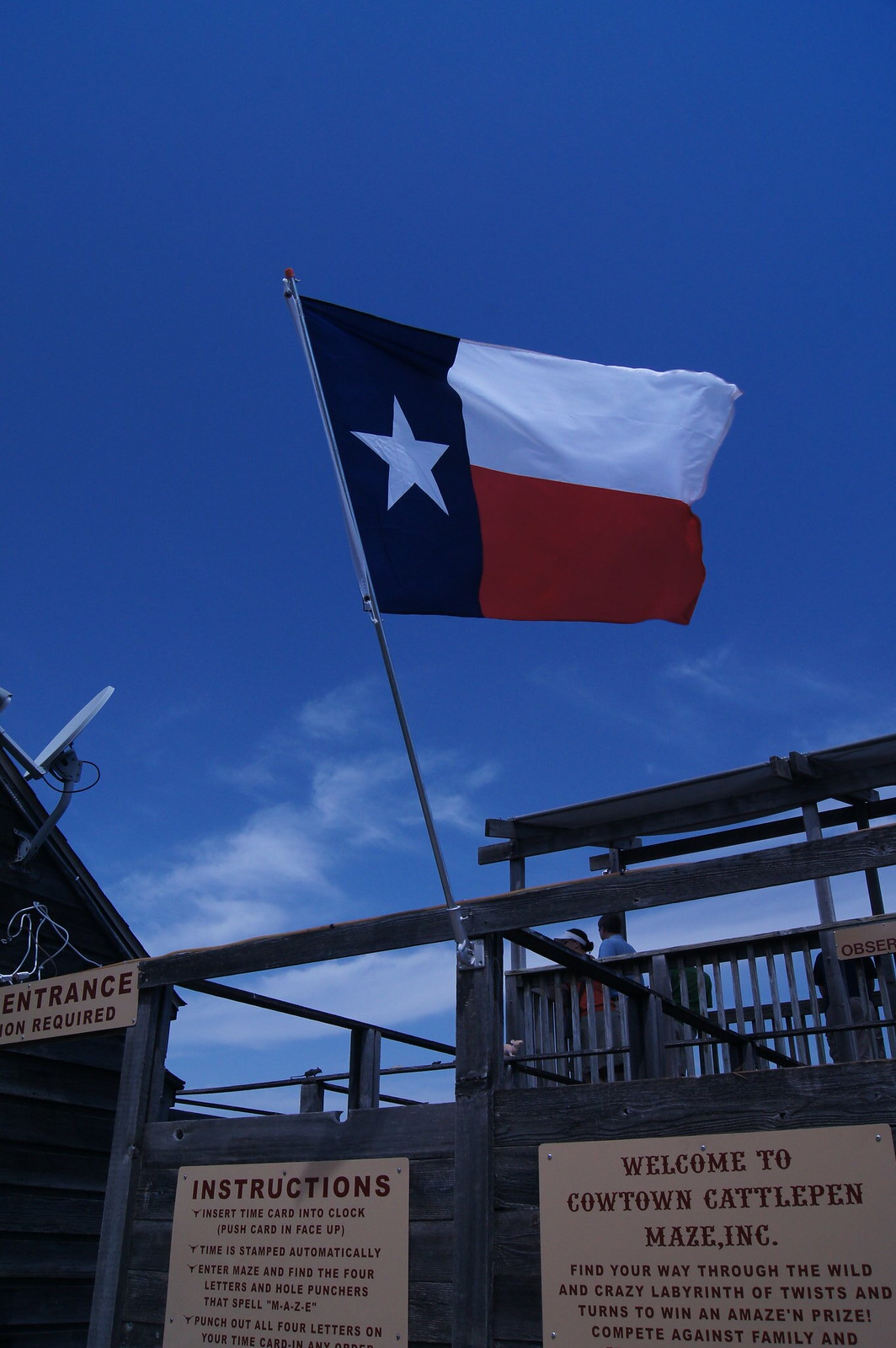This is a color photograph taken outside on a clear day with a deep blue sky. The focal point of the image is a large Texas flag prominently displayed on a long flagpole. The flag, featuring blue, white, and red horizontal stripes with a single white star on the blue stripe, is mounted on a wooden structure resembling a rodeo gate or a barn wall. 

Several signs are attached to the structure: the leftmost, partially visible, reads "Entrance, something required." The middle sign, labeled "Instructions," contains fine print directing participants to insert a time card into a clock, enter the maze, find four designated letters with hole punchers that spell "M-A-Z-E," punch the letters on the card, and so on, however, part of the text is not entirely clear. 

The rightmost sign declares, "Welcome to Cowtown Cattlepen Maze, Incorporated," inviting visitors to navigate through a wild and crazy labyrinth of twists and turns for a chance to win an amazing prize. The signs' text is in brown font on tan backgrounds. Though some small parts of the sign details are cropped out, it’s apparent that the photograph captures an entrance to an elaborate maze experience beneath the proud Texas flag.